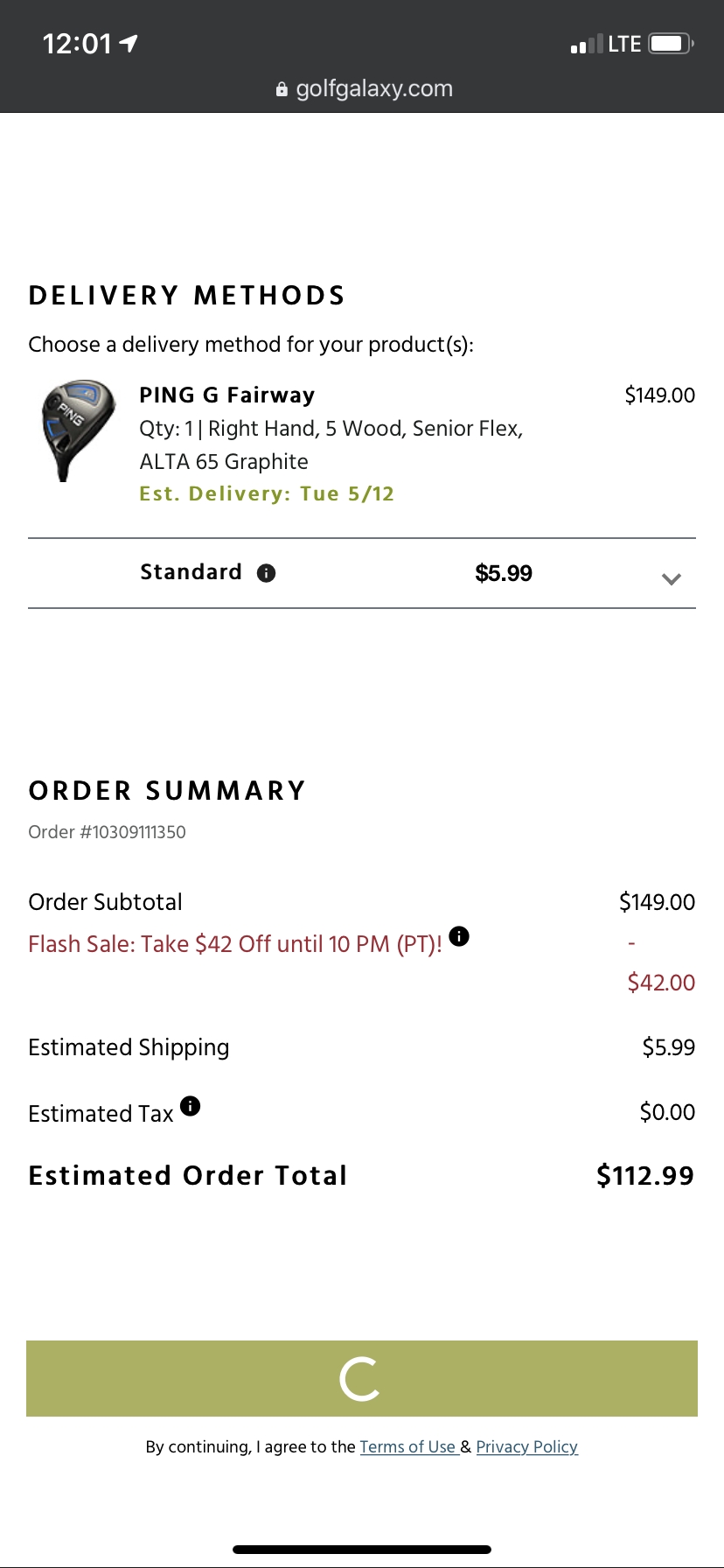This is a detailed caption for the screenshot from a cell phone:

"A screenshot from golfgalaxy.com, captured at 12:01 PM, shows the delivery options for purchasing a Ping G Fairway 5-wood golf club. The club is designed for right-handed players with senior flex and features an Alta CB 65 graphite shaft. The estimated delivery date is Tuesday, May 12. Priced at $149.00, a limited-time flash sale offers a $42 discount, reducing the total to $112.99. Standard shipping is listed at $5.99, with no additional tax added. The order summary includes order number 10309-111350. At the bottom of the page, links to the Terms of Use and Privacy Policy are visible, along with a 'Continue' button to proceed with the purchase."